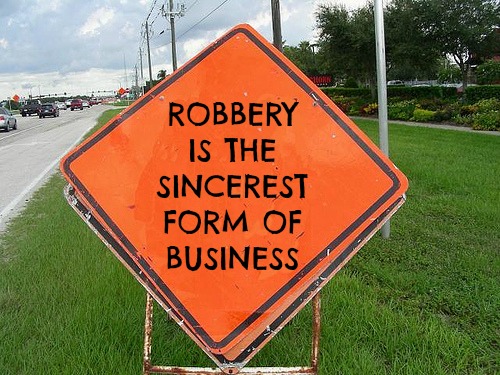This photo, taken outdoors on a cloudy day, features a fake road sign prominently displayed in the center, tilted diagonally like a caution sign. The sign is an orange diamond with a thin black border, held up by a rusty white post. In bold black lettering, the sign reads, "Robbery is the sincerest form of business." The scene is set on a lush expanse of bright green grass with a sidewalk to the right, accompanied by trees and flowers, and a row of light poles extending diagonally into the distance. To the left, a two-lane road with cars traveling in both directions can be seen, along with traffic lights further down the road. Overhead, power lines trace across the sky, which is filled with fluffy white clouds. The entire setting suggests it is part of a larger town or city.